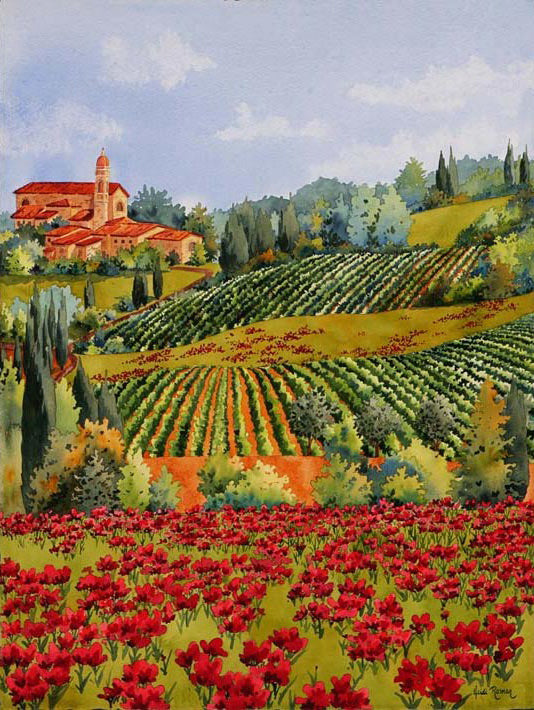The image is an artist's conception, possibly a painting, of a serene vineyard with the distinctive architecture of Italy or Greece. In the foreground, a lush field of blooming red flowers, resembling roses, adds vibrant color against the green ground. Tall, narrow shrub-like trees typical of the Mediterranean region dot the landscape. In the middle ground, rows of crops, likely grapevines, stretch in a linear pattern across the green side hills. Dominating the background is a majestic stone building with a red tile roof, featuring a spire and a small bell tower or turret—suggestive of either a winery, a farm building, or even a church. Surrounding the structure are more trees, and the scene is set against a beautiful skyline with light blue skies and patches of white clouds, and possibly distant mountains. The overall vista captures the peaceful and bountiful essence of a Mediterranean agricultural setting.